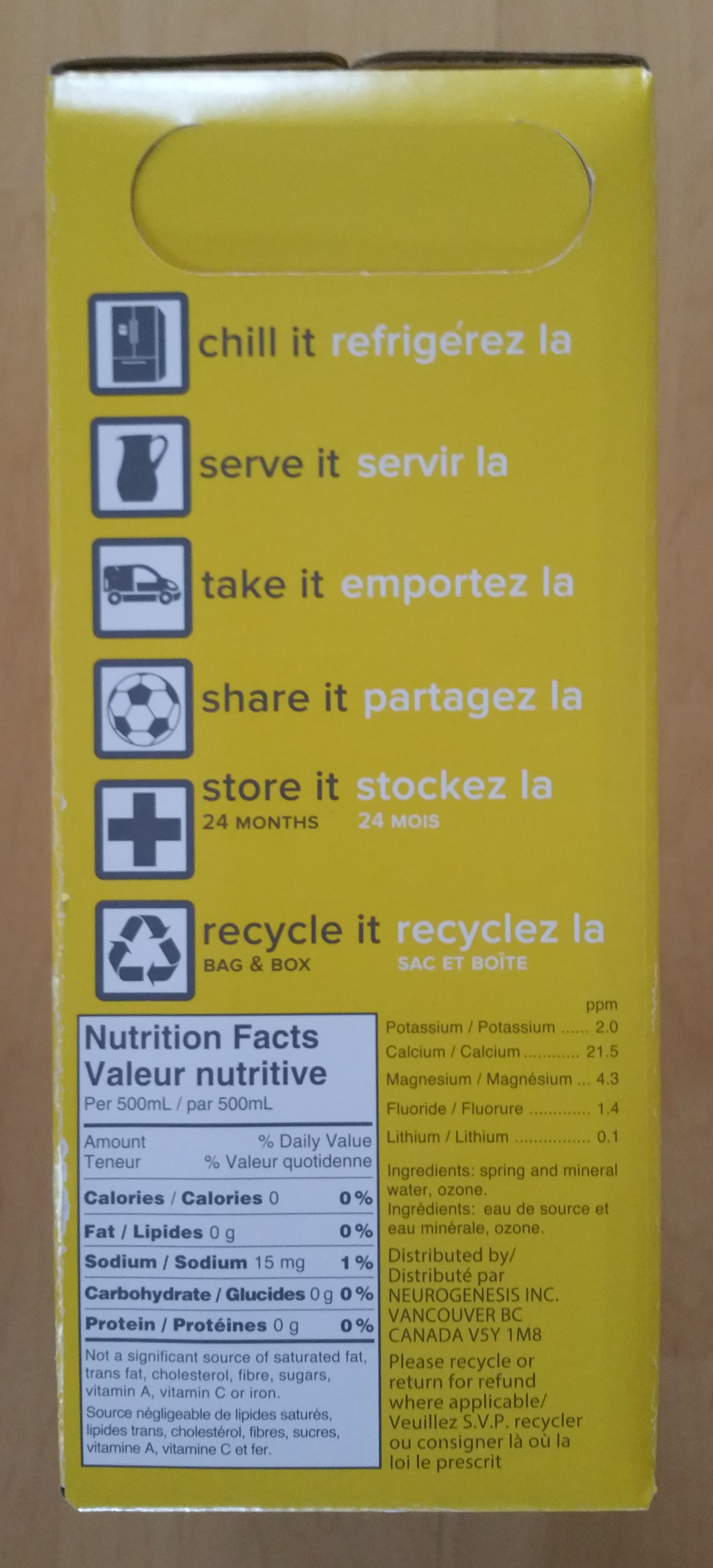The image showcases the side of a packaged box, specifically focusing on its nutrition facts label. The box, which is closed, has a distinct yellow background. Prominently positioned on the box is a rectangular-oval shape. Directly below this shape, there are action-oriented commands: "Chill it, serve it, take it, share it, store it, and recycle it." These phrases are accompanied by six corresponding emblems located to their left. To the right of the phrases, there is text in another language. 

On the left-hand side of the box, the nutrition facts are clearly listed, detailing the calories, fat, sodium, carbohydrates, and protein content. This information is presented on a white background, with additional text in another language immediately to the right of each nutritional element. Further to the right of the nutrition facts, there's additional information provided in short black text, enhancing the detail and usability of the label for consumers.